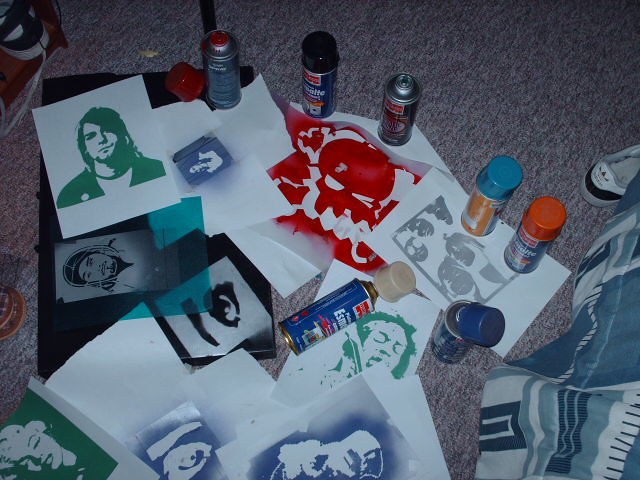In this overhead shot, the photographer captures a busy scene of artistic creativity unfolding on a gray-brown, short-fibered carpet floor. The room is strewn with numerous 8.5x11 white papers, each adorned with various spray-painted stencil sketches. Dominating the palette are shades of blue and black, with occasional splashes of red, green, and orange. Among these vibrant artworks, some recognizable images emerge: a man with a black beard, a green-painted man and woman, and a distinctive red skull. One particularly notable piece features a close-up of an eyebrow and eye, rendered in a cartoonish style. Adding to the scene’s creative clutter, there are six cans of spray paint, some with lids on displaying colors like red, black, light blue, royal blue, and orange, while a beige can lies at the center. Scattered around are a few empty papers, a black poster board, an Adidas sneaker, and what appears to be a blanket, indicating this moment of artistry might be taking place in someone's personal room or studio space.